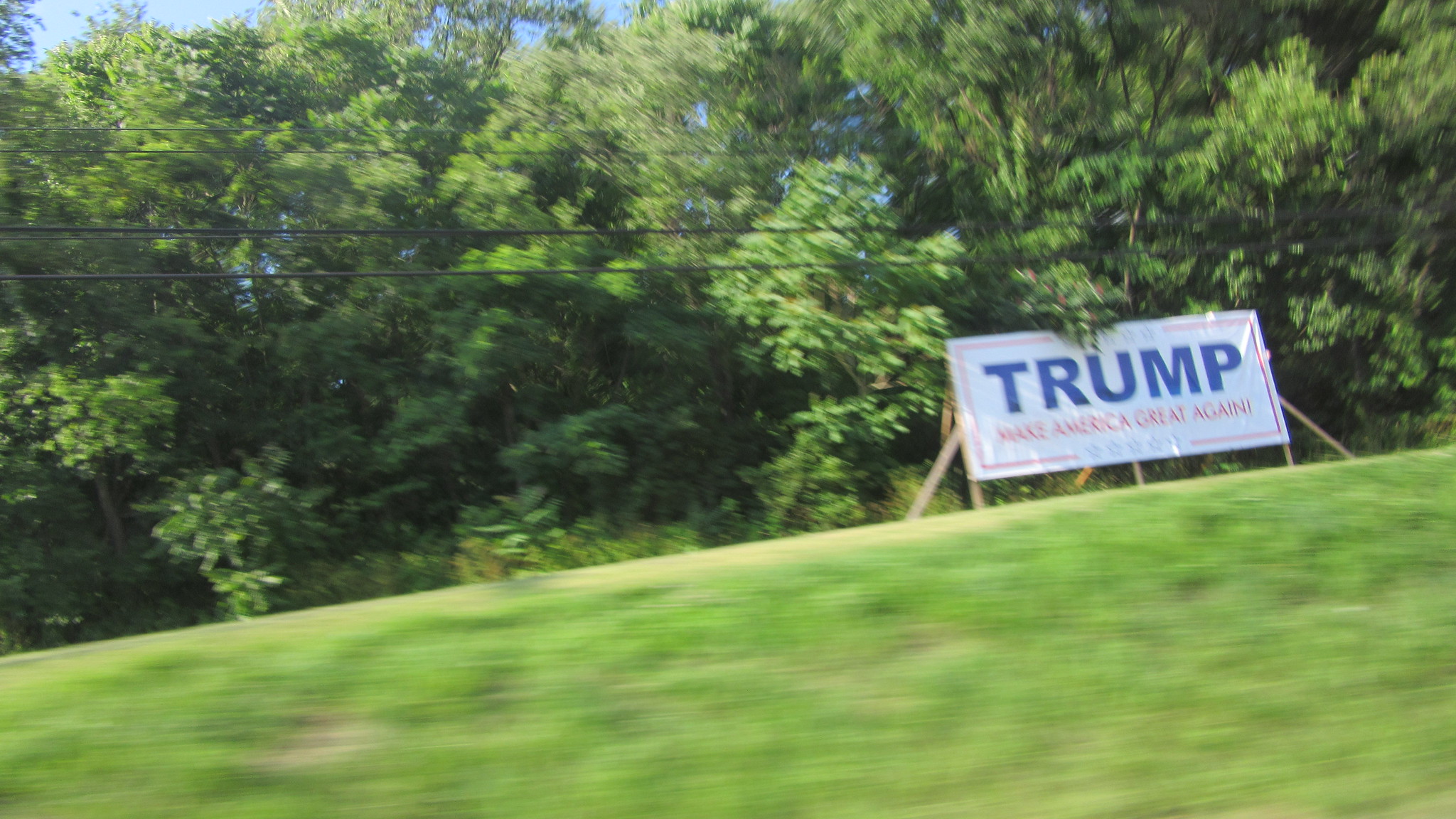In this color photograph taken from a moving car, a slight grassy hill adorned with a variety of tall, leafy trees forms the picturesque setting under a clear, blue sky. Towards the right-hand side of the image, prominently displayed on the slope, stands a large rectangular white sign with a thin red border. Blue letters spell out "TRUMP" at the top, while beneath it, in red letters, the slogan "MAKE AMERICA GREAT AGAIN!" is noticeable. The sign is slightly angled upwards and is supported by light-colored wooden beams anchored into the ground. Above the sign, several black power lines crisscross the bright sky. The image, captured on a sunny day, exudes a sense of motion, as the foreground blurs slightly, adding to the dynamic composition.